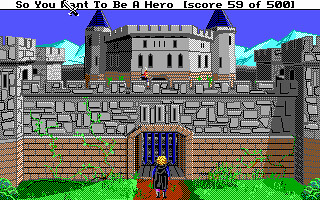This detailed and cleaned-up caption for the image would be:

"This is a screenshot reminiscent of an old-school video game, showcasing a medieval castle. At the top of the screen, text reads, 'So you want to be a hero,' accompanied by a score indicator, 'Score: 59 of 500,' in brackets. The castle, predominantly gray to depict stone construction, features a lower level made of red bricks. Green grass flanks an orange pathway leading up to the imposing structure. A small character stands at the entrance, which is barricaded by a blue, barred door, seemingly awaiting entry."